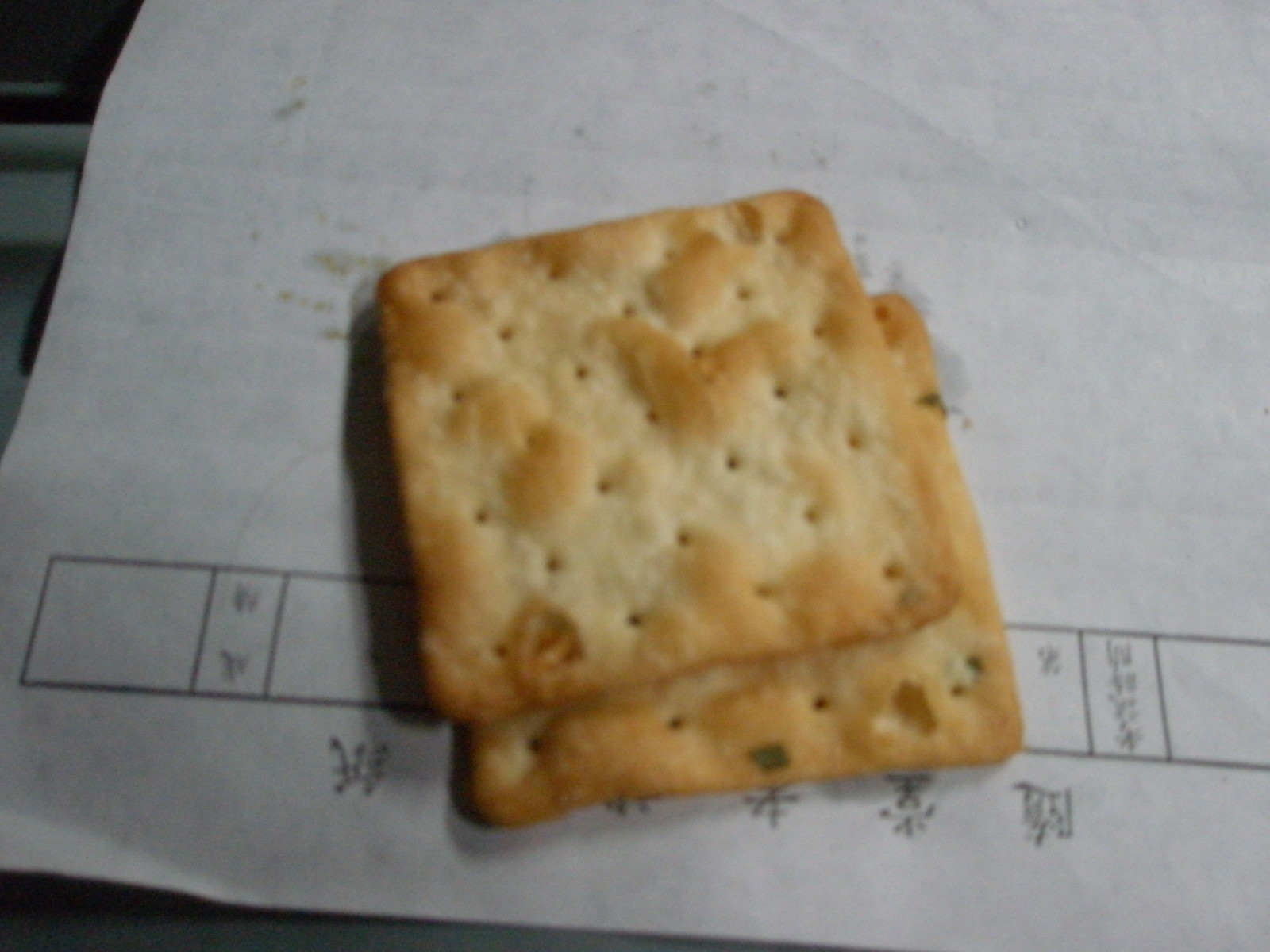The photograph features two light and crisp, square soda crackers, stacked one on top of the other. The crackers have a golden-brown hue and are perforated with small holes from baking, revealing airy pockets within the layers. The surface of the crackers displays a varied texture, with some areas puffed up and others flattened, indicating uneven baking. Small green specks, possibly bits of herbs or vegetables, are scattered across the crackers. They rest on a slightly dirty white piece of paper, adorned with what appears to be Chinese or Japanese characters and thin black lines. The paper itself shows signs of wear, with gray and yellow spots, and lies atop a dark, mottled surface.